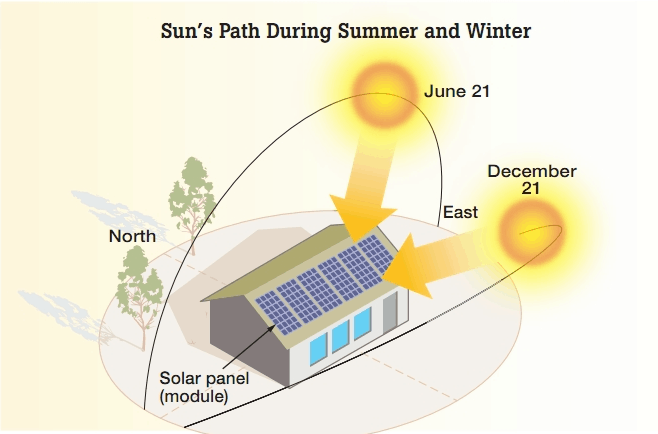The image illustrates the sun's path during summer and winter, depicted with an overhead view of a house with solar panels. At the very top center, black text reads "Sun's Path During Summer and Winter." Below the text, the house is shown with a top-down view, prominently featuring the roof adorned with six blue solar panels on the front side. The rest of the roof is light olive green, and the front facade of the house sports three blue windows and a dark gray door.

Above the house, two suns are illustrated: one at the top labeled "June 21," and another to the right labeled "December 21." Both suns are depicted as balls of orange and yellow with radiating light, and they each have arrows pointing towards the house, indicating the sun's path. Accompanying these labels, directional markers for east (near the right sun) and north (on the far left next to some green trees) are provided.

Surrounding the house, a creamy-colored circle or oval encompasses the ground area. Within this, additional annotations include a small black arrow pointing to the solar panels, captioned "solar panel (module)." A shadow cast by the house is oriented towards the north side, underlining the visual explanation of solar angles throughout the year.